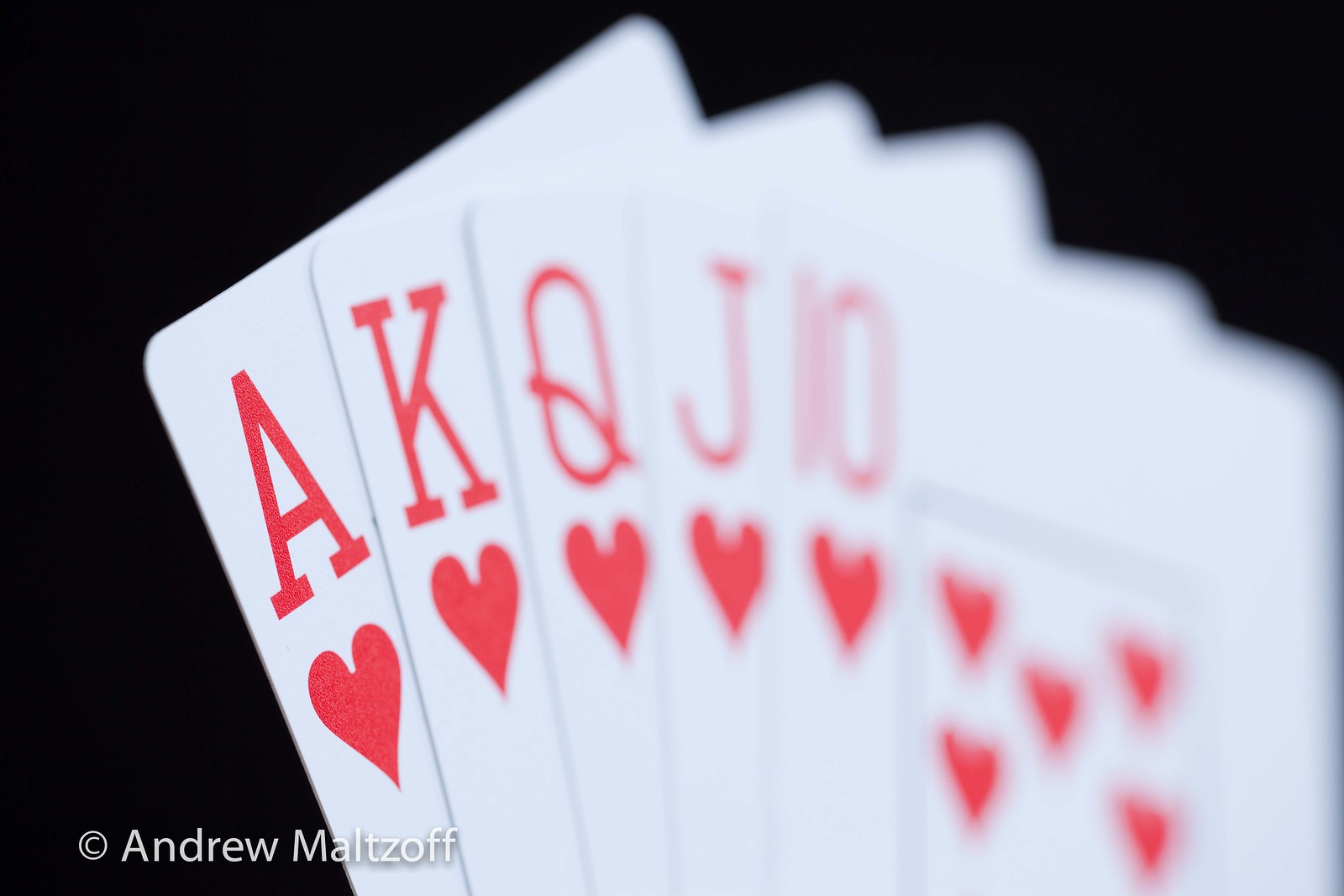The image features a set of five playing cards fanned out against a completely black background. The far left card is sharply in focus, progressively becoming more blurred towards the right. The cards displayed are from left to right: the Ace of Hearts, King of Hearts, Queen of Hearts, Jack of Hearts, and Ten of Hearts. While the Ace of Hearts is clear and detailed, the subsequent cards increasingly lose sharpness. By the time we reach the Ten of Hearts, the card is quite blurred, but a distinctive black rectangle with red hearts can still be discerned on its face. The bottom left corner of the image includes a white circle containing a white "C" and the name "Andrew Maltsoff," with "A" and "M" capitalized and the remaining letters in lowercase.